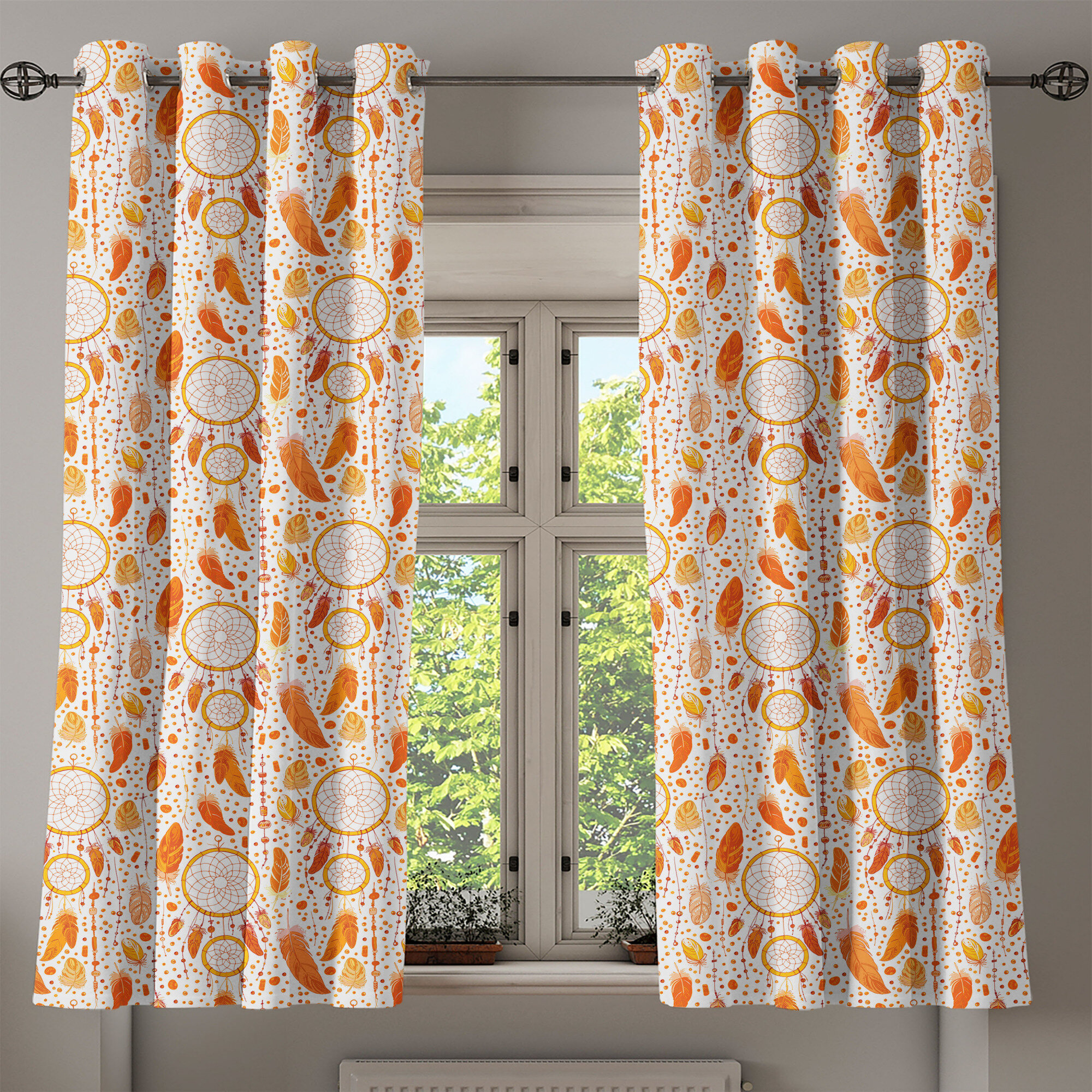This photograph captures a detailed view of a room with a distinctive window setting. The main feature is a white-framed window divided into four panes—two larger panes at the bottom and two smaller ones at the top, set within a pristine white wall. Vibrant curtains with a complex pattern of orange dreamcatchers, leaves, and feathers hang on a black curtain rod with round ends, creating a striking contrast with their white background. The curtains, split in the middle, showcase intricate designs reminiscent of symmetrical, floral motifs. Below the window, a white floorboard heater adds practicality to the scene. The windowsill holds a few pots with plants that appear to be withering, adding a touch of rustic charm and life to the setup.